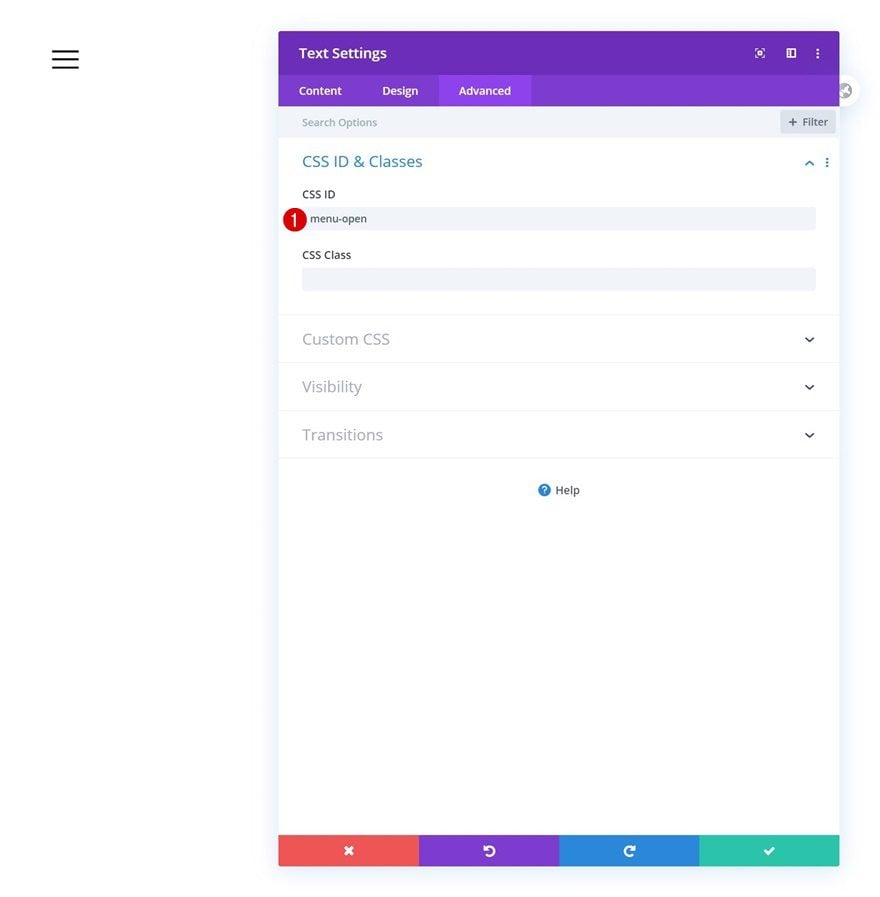The screenshot showcases an interface with a predominantly white background and a purple banner running across the top. On the left side of this banner, the text "Text Settings" is displayed in white. On the far right, there are three clickable icons, including a three-dot menu that usually indicates additional settings or options.

Directly below "Text Settings," there are three tabs labeled "Content," "Design," and "Advanced," with the "Advanced" tab currently selected. Beneath this section, there is a search bar on the left and a "Filter" button on the far right.

Further down, the interface displays options for "CSS ID" and "Classes" in blue font, with a collapsible caret icon on the right that allows users to expand or hide this information. There is another three-dot menu next to this caret icon.

Underneath the CSS options, a field labeled "CSS ID" contains the text "menu open," accompanied by a circular icon with the number one to its left. Below this, there is another field labeled "CSS Class."

The text "Custom CSS," "Visibility," and "Transitions" appear in a grayed-out font below the CSS fields, each accompanied by a collapsible caret icon, indicating that these sections are currently closed.

At the very bottom of the interface, there are four options centered within the screen: on the far left, an "X" icon; next to it, an "Undo" icon; followed by a "Redo" icon; and on the far right, a check mark. These options presumably allow users to exit, undo, redo, or save their changes, respectively.